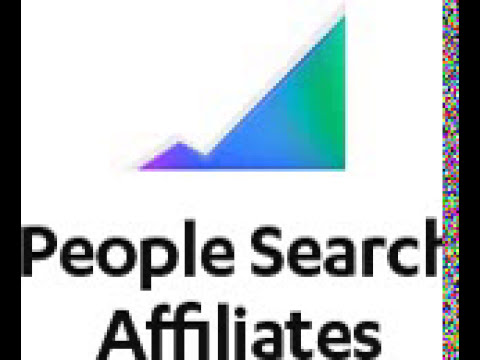The image depicts a low-resolution corporate logo against a simple white background. Central to the design is a graphic composed of two intersecting triangles. The larger triangle lies on its side, transitioning from blue to green, and features a unique, jagged edge that slopes down, briefly slopes up, and then slopes down again, creating a small peak at its bottom. This gradient triangle overlaps with a smaller purple triangle positioned at its lower left. Below this graphic, in bold black text, the words "People Search Affiliates" are prominently displayed. The image is framed by black lines running vertically down its sides, with an additional vertical bar on the right side showcasing a series of multicolored static dots, adding a dynamic touch to the otherwise straightforward design.